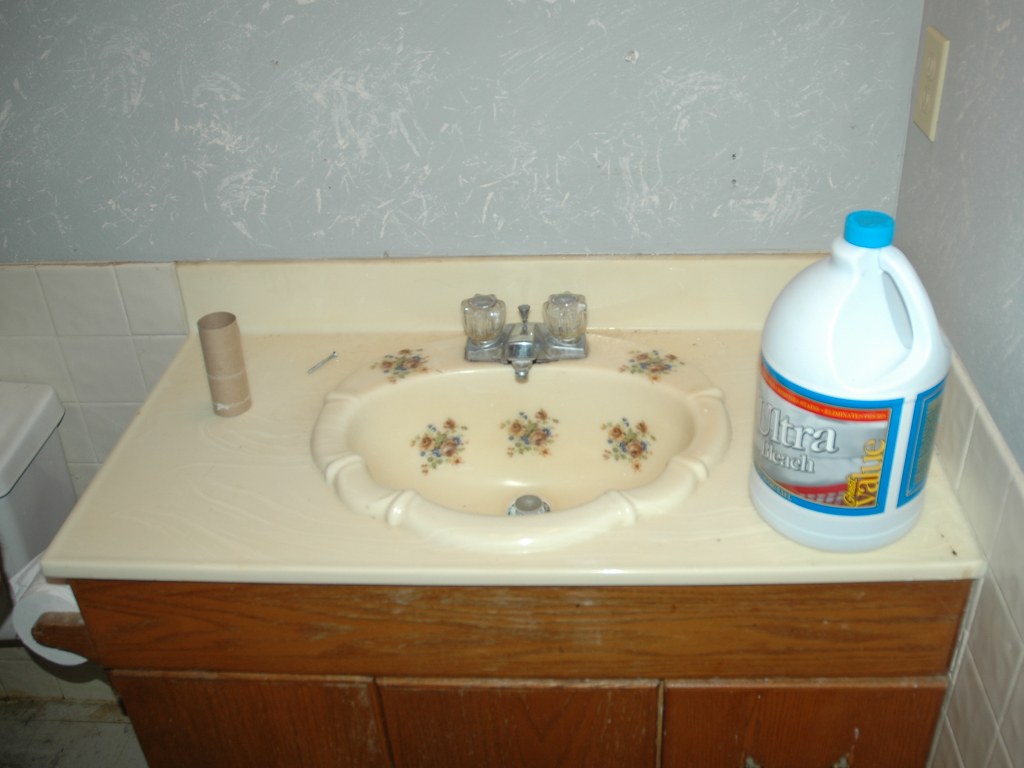This image captures a detailed view of a bathroom corner, featuring a peach-colored basin frame. The upper half of the bathroom walls is adorned with dusty blue wallpaper with white marbly patterns. On the left side of the basin top, there's a finished toilet roll and a nail resting on it. The basin itself is decorated with beautiful flower stickers: two are positioned on the top right, one on the top left of the taps, and three are inside the basin.

To the right of the basin, there's a 5-liter bottle that appears to contain bleach, distinguished by its light blue label and matching blue lid. Above the bleach bottle, a wall socket is installed. The lower half of the wall is tiled with very small squares, creating a neat, geometric pattern. The basin is mounted on a round cupboard below, adding both functionality and a touch of elegance to the bathroom's corner.